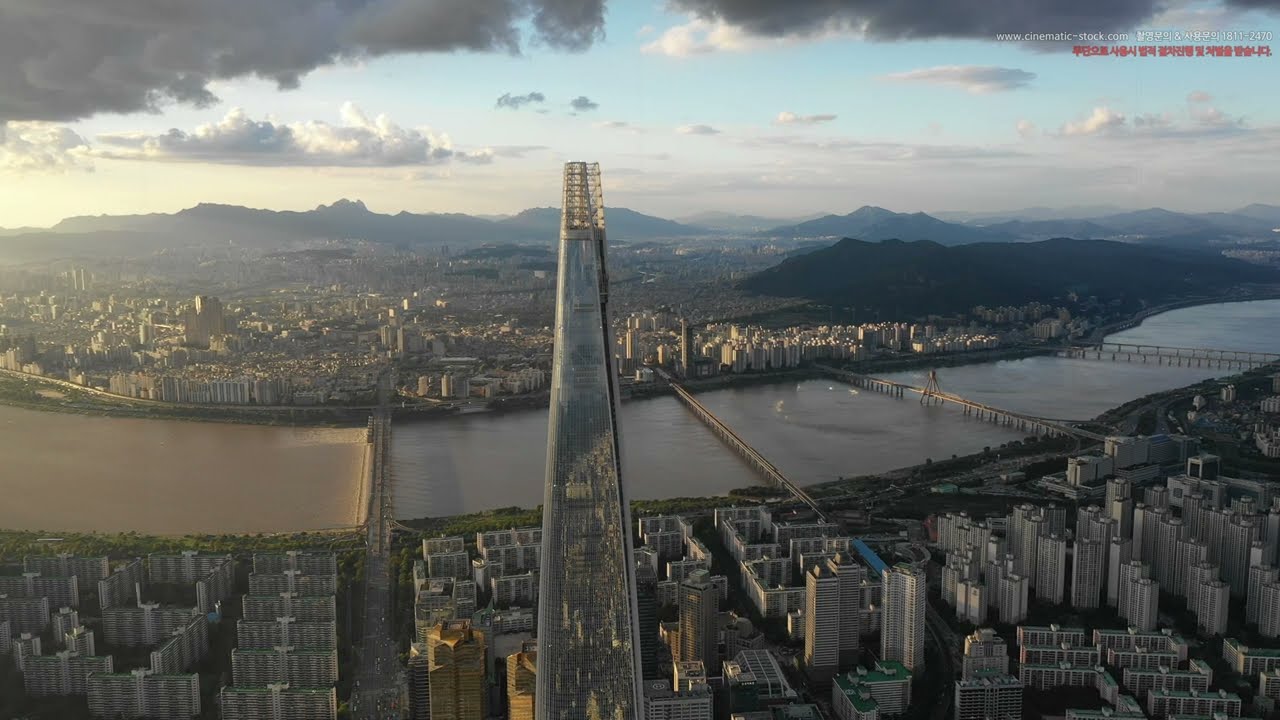This color aerial photograph, taken from a high vantage point, likely a drone, captures an expansive view of St. Louis with a detailed, realistic style. Dominating the central image is the iconic Gateway Arch, which appears to curve gracefully towards the camera from the lower part of the photograph, creating a focal point much closer than any other elements. The Mississippi River, with its characteristic brown, muddy hue, runs horizontally from the right to the left, intersected by four distinctive bridges, linking the city's two sides. The cityscape beneath and beyond the Arch is populated with tall, high-rise buildings arranged in fairly regular patterns, with commercial areas and wide streets. Further in the background, the dense cluster of buildings transitions into a congested urban sprawl. Distant mountain ranges rise on the horizon under a mix of blue skies and dark, brooding clouds. The upper right corner of the image contains a text overlay reading "www.cinematicstock.com" in white script, accompanied by Asian lettering in both white and red fonts, enhancing the image's detailed composition.